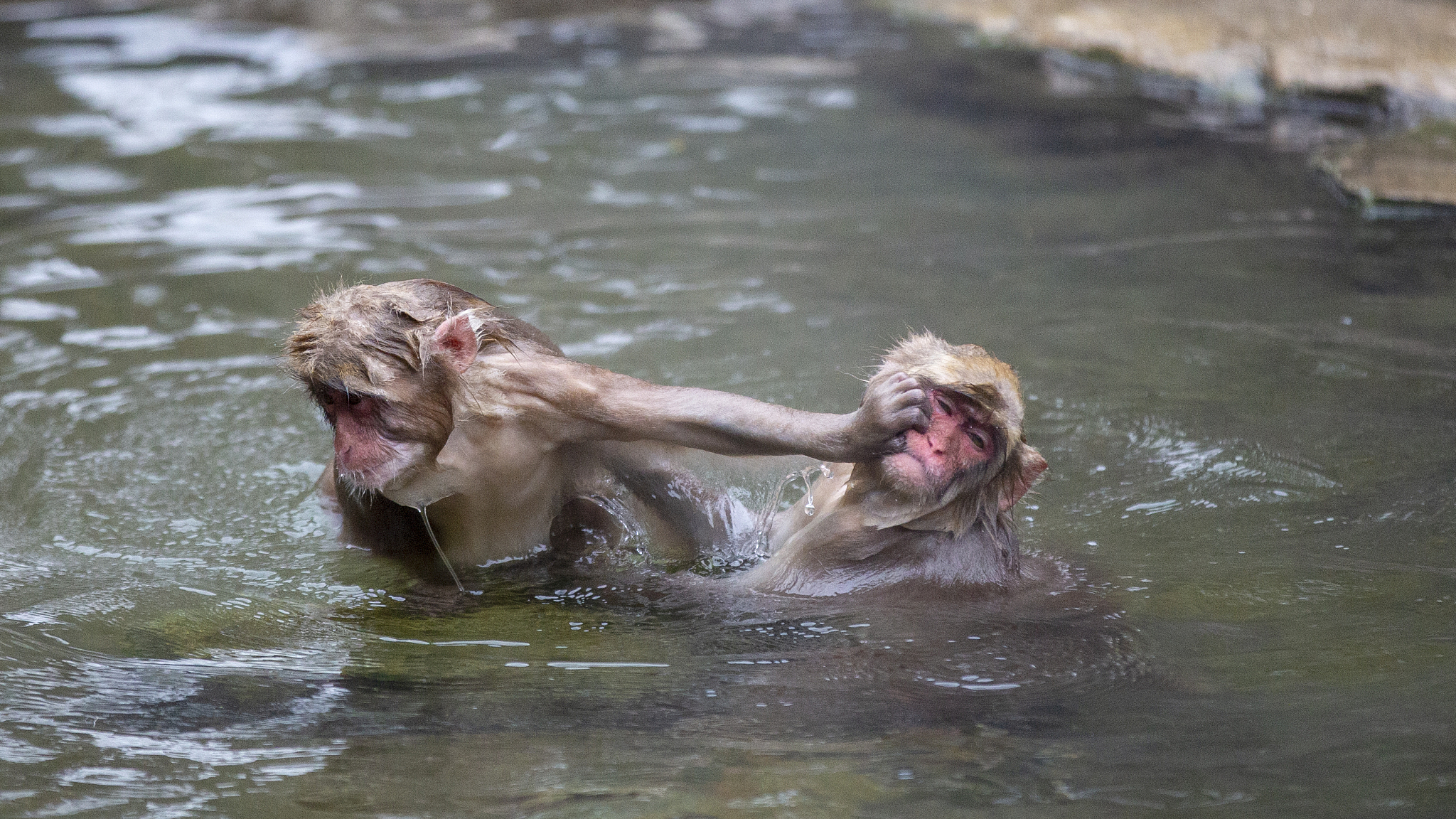This horizontal outdoor photo captures two small baboons immersed in greenish-brown water. The baboon on the left, facing slightly away from the camera, is forcefully pushing its hand against the cheek of the other baboon, who faces the camera with a displeased expression. Both baboons are soaking wet, with water dripping off their bodies, indicating recent splashing and thrashing. Their lower bodies are submerged, and only their upper bodies and heads are visible. The shallow water they are in is disturbed, creating noticeable waves, and rocks are visible both beneath the water’s surface and in the background. The interaction between the baboons could be interpreted as playful or confrontational.